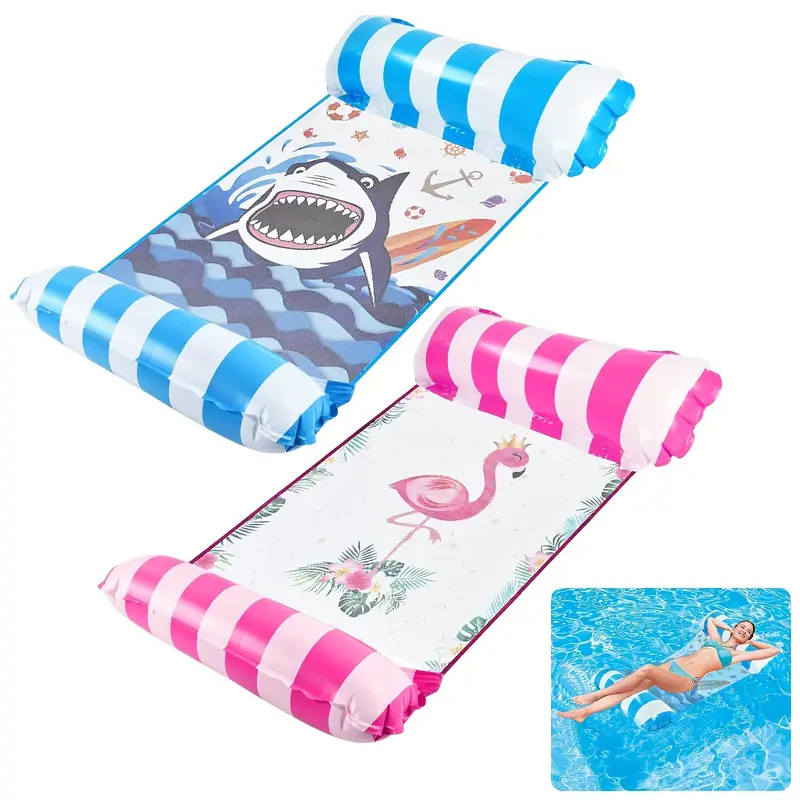The image comprises three stacked photographs, unified by a pool and inflatable pool toy theme. The top picture features a blue and white striped inflatable pool raft with a fabric section in the middle depicting a cartoon shark, resembling the character from "Finding Nemo". This raft includes inflatable pillows on each end and is designed so that the middle section is submerged in the water. Below it is a pink and white striped raft with a fabric insert showing a cartoon flamingo wearing a golden crown, standing on one leg amidst green tropical palm fronds. The bottom right corner of the composite image shows a woman relaxing on the blue and white raft in a turquoise blue pool, further emphasizing the aquatic leisure theme.